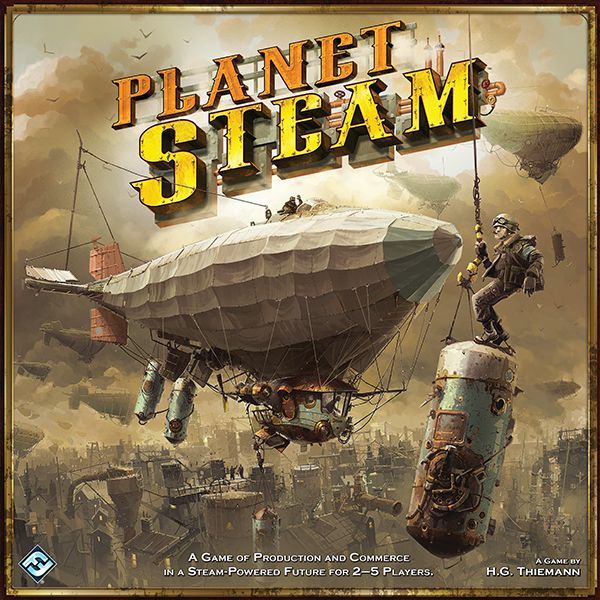The image is a detailed color illustration with a striking steampunk theme, presented in a square format. Central to the composition is a Zeppelin-like airship with a pointed nose facing right. The airship features a beige body and a hanger structure beneath it, from which various items dangle. Overlaid on the image, in antique typography, are the words "Planet Steam"—'Planet' in bold orange and 'Steam' in bold yellow, both words angled and in all capital letters.

Positioned to the right of the image is a man dressed in military uniform, standing atop a hanging, bomb-like cylindrical structure, gripping a cable attached to the airship. The scene portrays a dark, cloudy sky filled with grayish-brown clouds, while a few beige-tone birds float around, enhancing the aerial perspective. Below, the cityscape, painted in grayish-brown hues, sprawls out, adding depth and context to the illustration.

In the foreground at the bottom, white text reads: "A game of production and commerce in a steam-powered future for two to five players." Additionally, there is a small black diamond shape with the letter "F" on the bottom left, and on the bottom right, the text reads "A game by H.G. Thiemann." The overall atmosphere is suggestive of military and warfare, underscoring the game's adventurous and strategic elements.